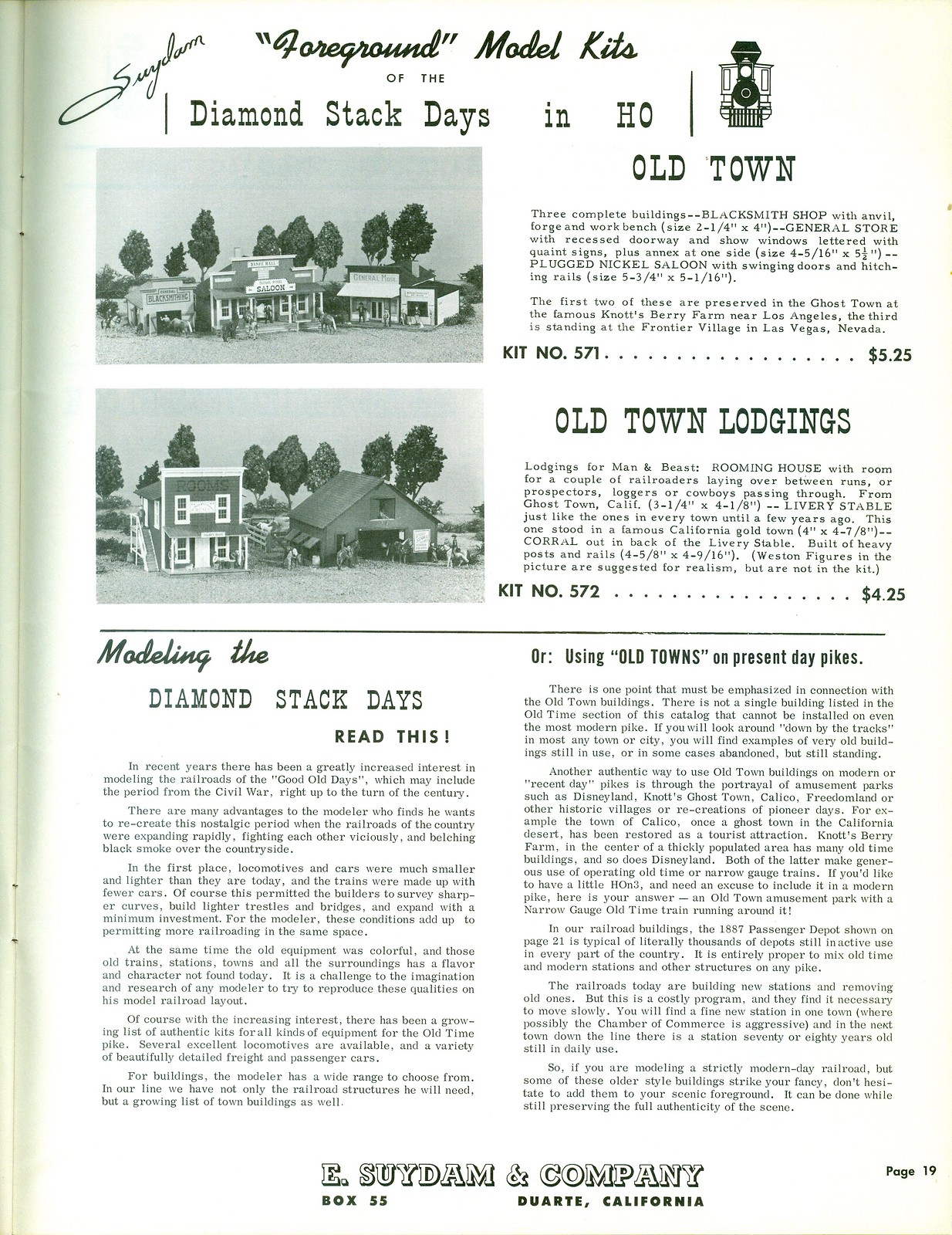This image features a page from a catalog, presented on a white background. The top half of the page displays the title "Foreground Model Kits of the Diamond Stack Days in H.O. Old Town" in black letters. Below this are two black-and-white photos arranged vertically, showcasing detailed model kits of vintage buildings. The first image depicts "Old Town," which includes three complete buildings: a blacksmith shop with anvil, forge, and workbench; a general store; and the Plug Nickel Saloon. This kit, identified as number 571, measures approximately 2.25 by 4 inches and is priced at $5.25. The second image shows "Old Town Lodgings," featuring a rooming house, livery stable, and a corral. This kit is number 572 and costs $4.25. The bottom of the page contains text about modeling the Diamond Stack Days, emphasizing their historical context and application in model railroads. The page concludes with the company details: E. Soydam and Company, Box 55, Duarte, California.